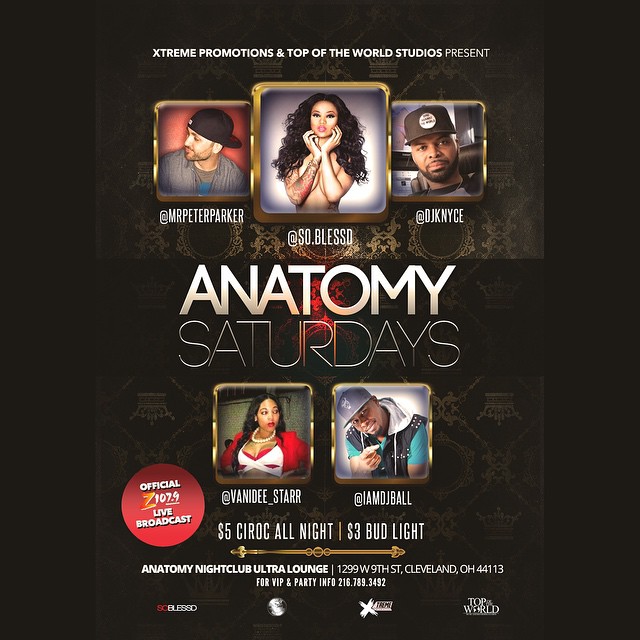The image is a large square poster with a predominantly solid black background, featuring promotional content for an event called "Anatomy Saturdays" at the Anatomy Nightclub Ultra Lounge, located at 1299 West 9th Street, Cleveland, Ohio. 

At the top, white text reads "Extreme Promotions and Top-of-the-World Studios Present." Below this header, there are three square thumbnail photos, each with a gold border. The left photo shows a man wearing a backwards black ball cap, looking off toward the left, identified as @Mr.PeteParker. The middle photo is of a woman, seemingly without a shirt and with tattoos on her right arm, with her hands up to her chin, labeled @So.Blessed. The right photo features a man with short, trimmed black facial hair and a hat, looking directly at the camera, noted as @DJKNice. 

In the center of the poster, large white bolded text states: "Anatomy Saturdays" in all capital letters. Below this central text are two more square thumbnails with gold borders. The left image depicts a woman in red and white attire, looking to the right, tagged as @Vanity_Star. Next to her, a man in a black hat, blue t-shirt, and black vest, looking at the camera, is labeled @IAmDJBall.

Further down, the poster promotes $5 Ciroc drinks and $3 Bud Light available all night. An official seal indicates that this event includes a live broadcast by Z 107.9. A gold arrow points to the event's details, which are written in white text, including information for VIP and party inquiries with a contact phone number.